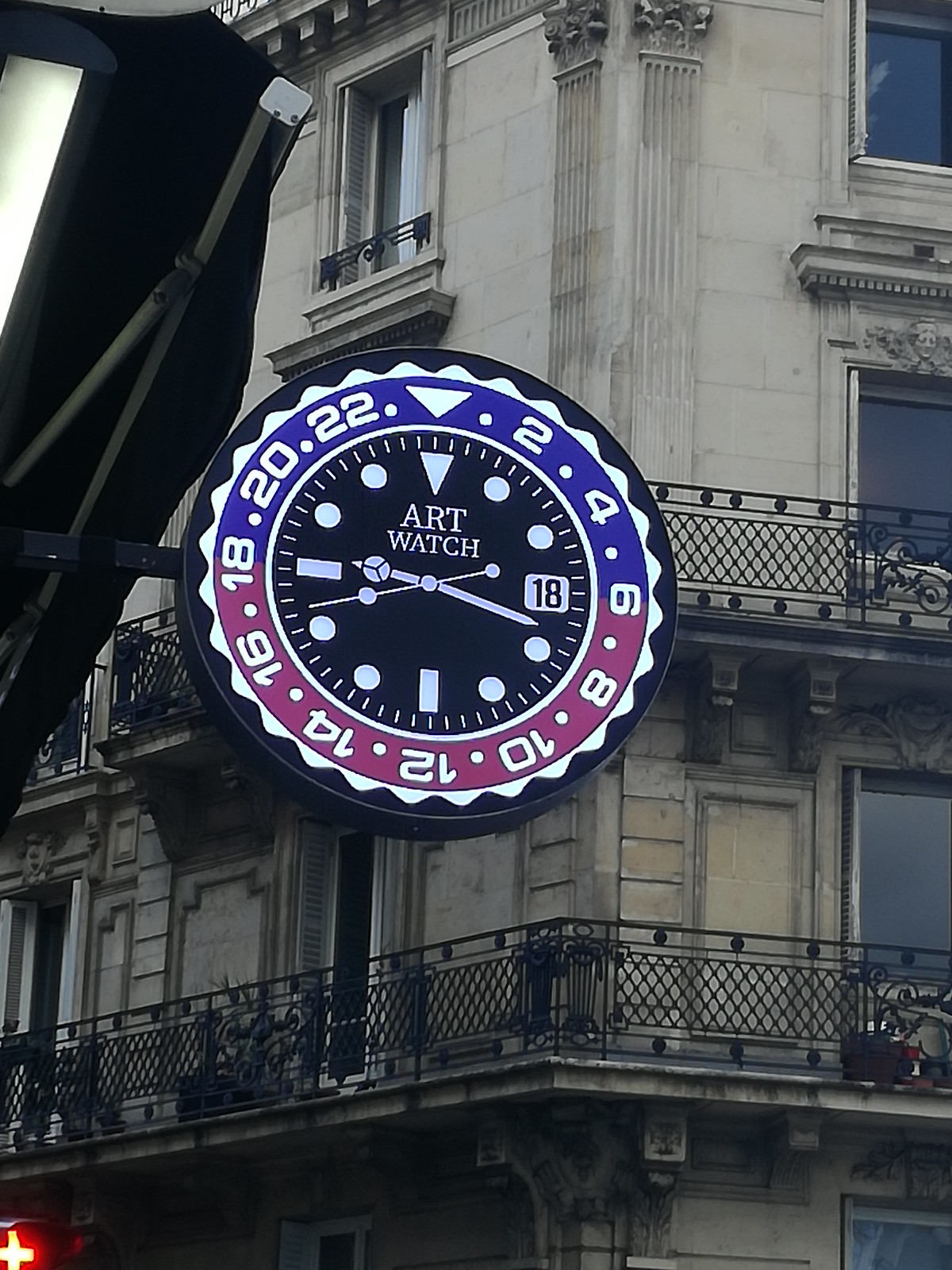The photograph captures an old, intricately decorated, multi-story brick building, featuring classic rectangular windows and a large black and colorful analog clock mounted on its corner. This distinctive timepiece, almost spanning the height of one story, displays a unique military time format with numbers following a pattern of odd numbers from 2 to 22. The top half of the clock's trim is blue, and the bottom half is red, with light blue dots representing the traditional number positions. The central part of the clock, where the silver minute and hour hands are located, is black with the words "Art Watch." Adding to the scene is a notable detail—the presence of a Swiss flag in the lower left-hand corner, hinting at the potential location of this vintage architectural setting. The clock indicates a time of 9:20.